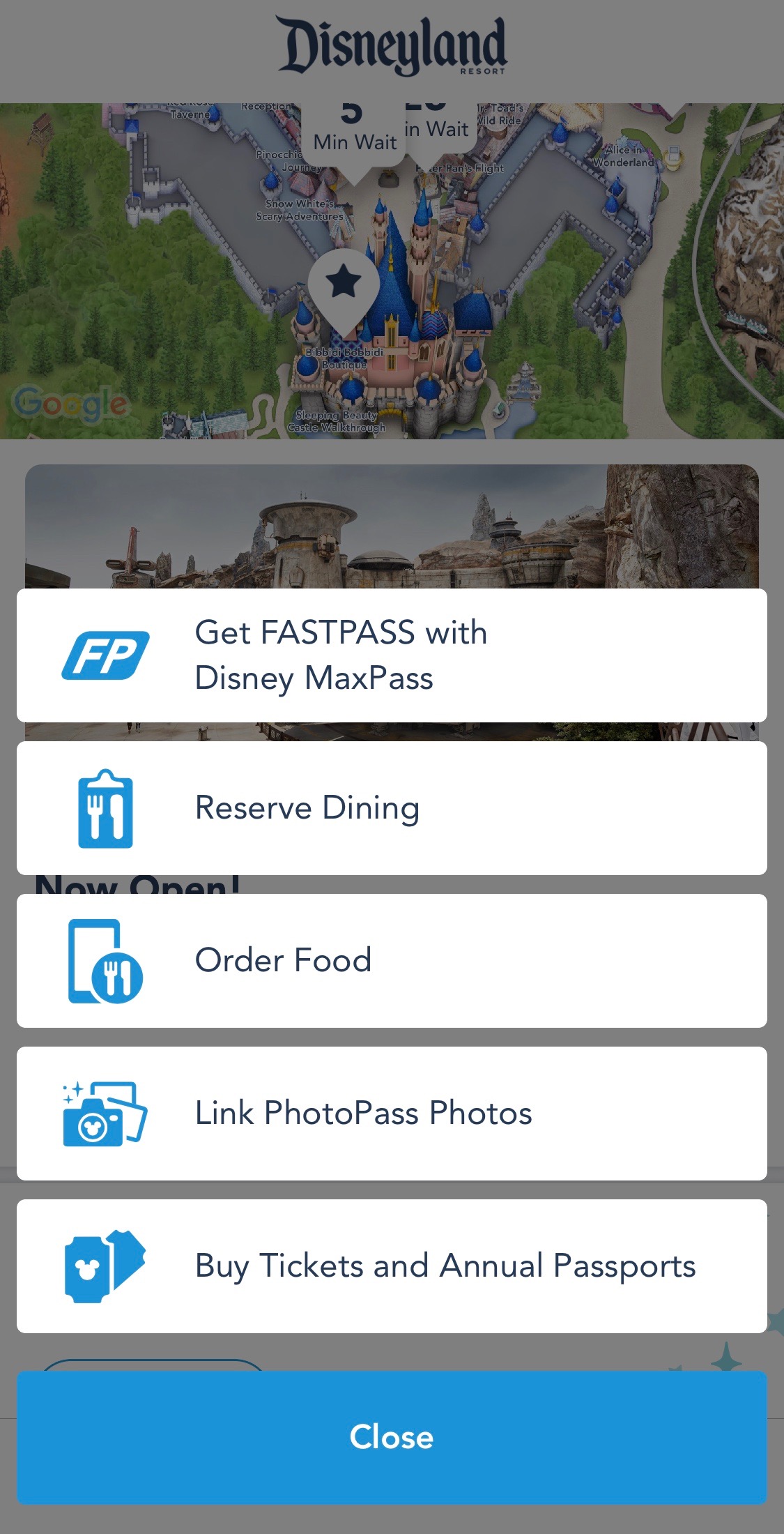This image displays a cell phone screen showing a Disneyland webpage. At the very top, there is a white triangle with the word “Disneyland” prominently displayed. Directly beneath this triangle, there is a tab labeled “Minute Wait,” and another identical tab follows it. 

Below these tabs, the screen features a detailed map of Disneyland, easily recognizable by the iconic castle illustrated at the center. The castle is marked with a teardrop emblem featuring a black star.

Moving further down, there are additional white triangles stacked vertically, each containing distinct blue icons. The first icon, labeled "FP" in white letters, is uniquely shaped like a stretched-out rectangle, resembling a parallelogram. The accompanying text reads, “Get Fast Pass with Disney MaxPass.”

Next, a blue emblem resembling a fork laid on a clipboard, signifies the "Reserve Dining" option. Below that, another circular icon displays a fork and knife above a rectangle, indicating the "Order Food" feature.

Following that, there’s a camera icon with overlapping photo frames in the background, labeled “Link PhotoPass Photos.” Finally, there is an icon depicting blue tickets adorned with Mickey Mouse emblems, which leads to the “Buy Tickets and Annual Passports” option.

At the very bottom, a blue rectangle labeled “Close” serves as an exit button for this section of the webpage.